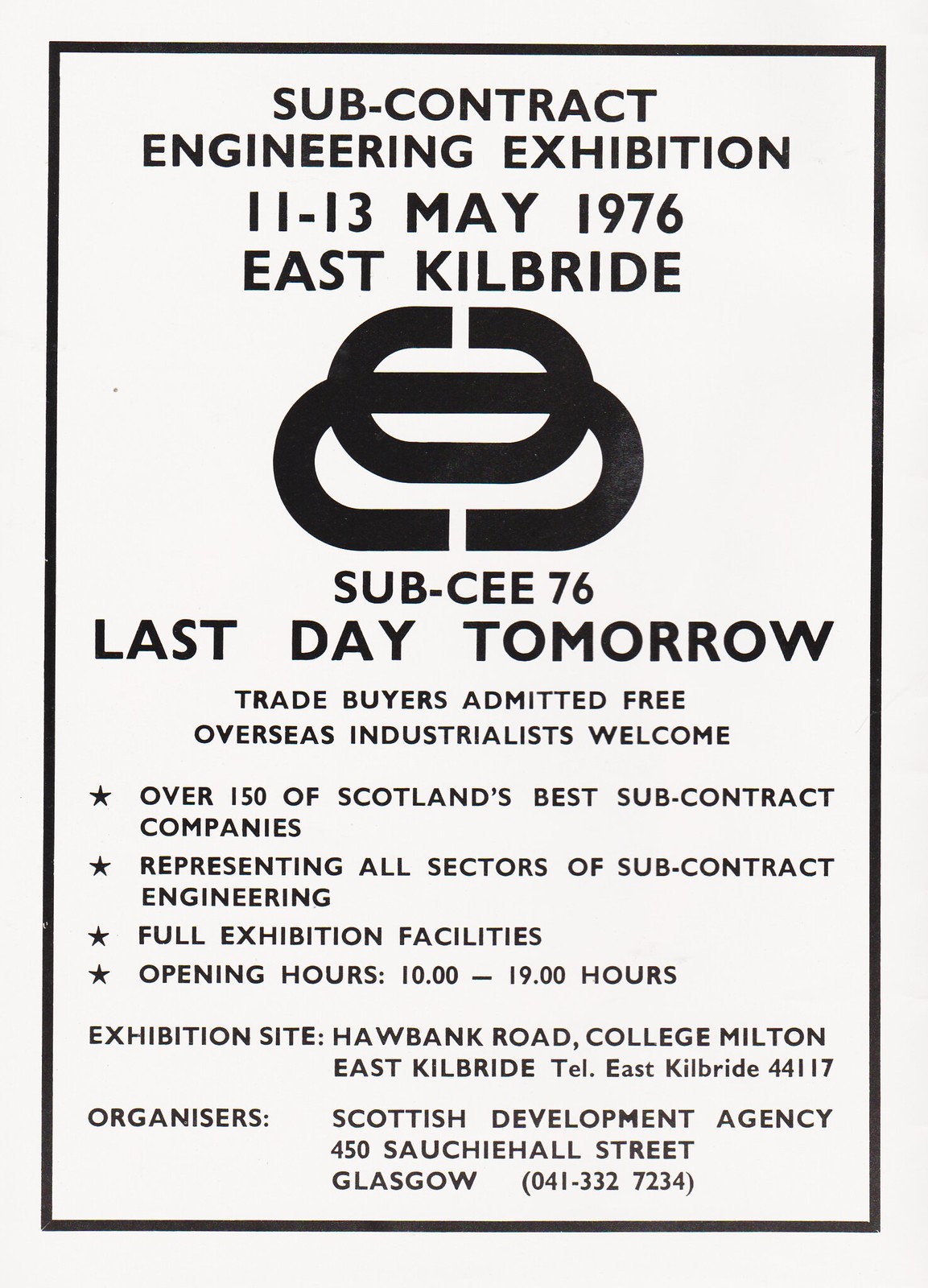The image is a tall, off-white exhibition flyer with a thin black border. Centered at the top in bold black capital letters, it reads: "SUB-CONTRACT ENGINEERING EXHIBITION 11-13 MAY 1976 EAST KILBRIDE." Below this text, in the middle of the flyer, are two overlapping 'C' symbols—one facing up, the other down. Beneath these symbols, the text continues: "SUB C-76, LAST DAY TOMORROW."

The flyer provides various details in black capital letters with small black stars next to each point on the left side. The starred details are as follows:
- "Over 150 of Scotland's Best Sub-Contract Companies,"
- "Representing All Sectors of Sub-Contract Engineering,"
- "Full Exhibition Facilities,"
- "Opening Hours 10-1900 Hours."

At the bottom, the flyer lists the location and contact information: "Exhibition site: Hawbank Road, College Milton, East Kilbride, East Kilbride 44117. Organized by the Scottish Development Agency, 450 Sauchiehall Street, Glasgow, 041-332-7234." 

Additionally, other highlights on the flyer state: "TRADE BUYERS ADMITTED FREE" and "OVERSEAS INDUSTRIALISTS WELCOME." The main text at the top is noticeably larger than the informational text at the bottom.